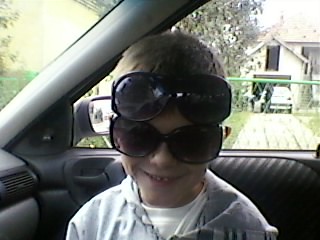In this photo, a young boy, approximately eight to ten years old, sits in the passenger seat of a car, smiling. The child's short sandy blonde hair peeks out from under two sets of large, bubble-style sunglasses—one on his face and the other perched on his forehead. He wears a button-up shirt over a white t-shirt, and the car's interior features a mix of light and dark gray tones. The background reveals a sunny outdoor scene with a green fence, white house, and a concrete driveway with green trees visible. Additionally, another vehicle and a garage can be seen behind the boy, adding to the suburban setting. The passenger side mirror is also visible within the frame. The image captures a playful moment, with the boy's dual sunglasses adding a touch of whimsy to the scene.